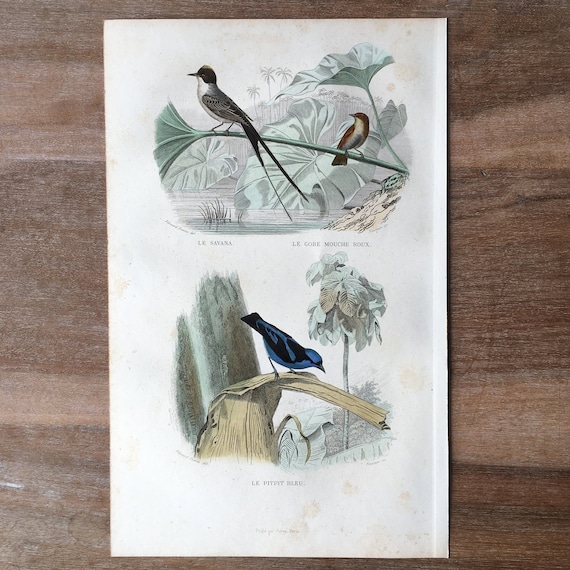The image depicts a photograph of an aged, slightly splotchy page from an old field guidebook or similar illustrative work, placed on a wooden tabletop. The page features two exquisitely detailed pencil drawings or paintings of birds in natural settings. The upper drawing showcases a striking scene of a black bird with a long, scissor-shaped tail and a smaller bird, both perched on a large, lily pad-like leaf stem above water, with faint grey palm trees in the background. The black bird boasts a white chest resembling a helmet and appears to be the male, while the smaller bird with a similar white chest might be the female. Below this, the second illustration presents a blue and black bird intently watching what could be a small insect, perched on a wooden branch or dried leaf, set against a background featuring large leaves. The text on the page, though partly blurry, includes titles such as "La Savanna," "Le Gaube Mauchereau," and "Le Petit Bleu,” adding a layer of historical authenticity to the document.